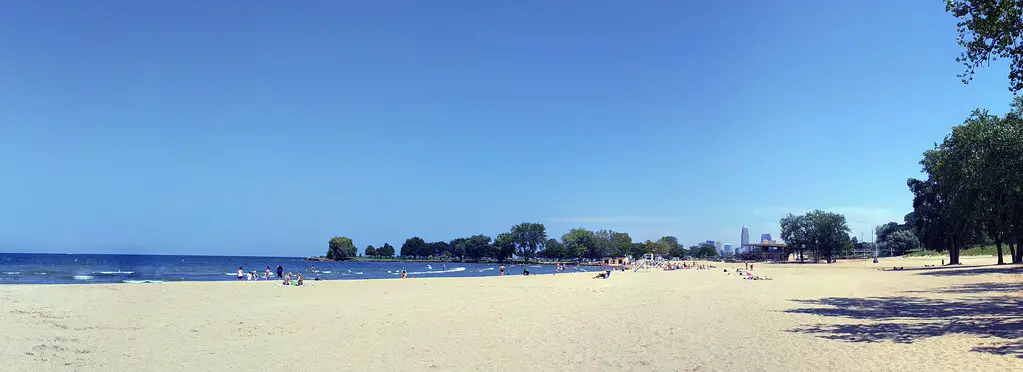This panoramic image captures a vibrant beach scene on a bright, sunny day with a brilliant blue sky dotted by a few wispy white clouds in the far-right background. The pristine white sand stretches expansively across the foreground, illuminated by the clear midday sun, casting dappled shadows from clusters of green trees on the right. The dark blue ocean, located to the left, contrasts beautifully with the lighter blue sky, dotted with white waves crashing onto the shore. Numerous beachgoers can be seen, some lounging on the sand while others frolic in the water. In the far background, both to the right and center, a green tree line extends, following the coast's gentle curve, creating a picturesque bay. Additionally, tiny city skyscrapers dot the distant center horizon, hinting at a nearby metropolitan area. This idyllic scene beautifully encapsulates a lively yet serene beach day.